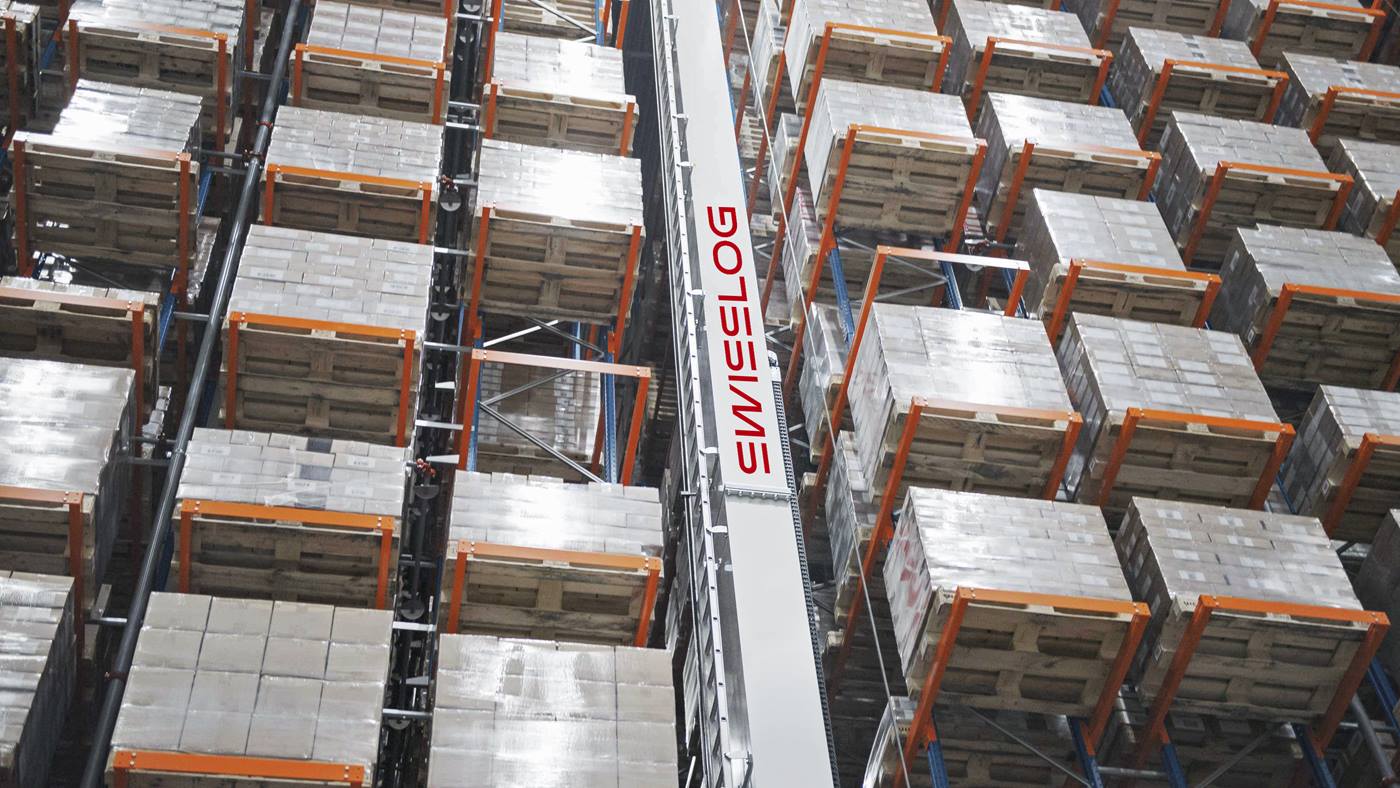This aerial photograph captures a detailed view of an industrial warehouse facility, specifically a sophisticated shipping area. Dominating the center of the image is a large white wall that acts as a horizontal divider, bearing the name "Swisslog" in prominent, sinewy red letters. Flanking either side of this wall are numerous steel towers with a yellowish-orange hue, uniformly organized into rows. Each tower holds an array of pallets, which are neatly stacked with square, flat stones or cement-like blocks, many of which appear to be covered with plastic sheets, suggesting a readiness for shipping. The heavy-duty machinery and overall layout indicate a highly organized environment tailored for industrial shipping purposes.